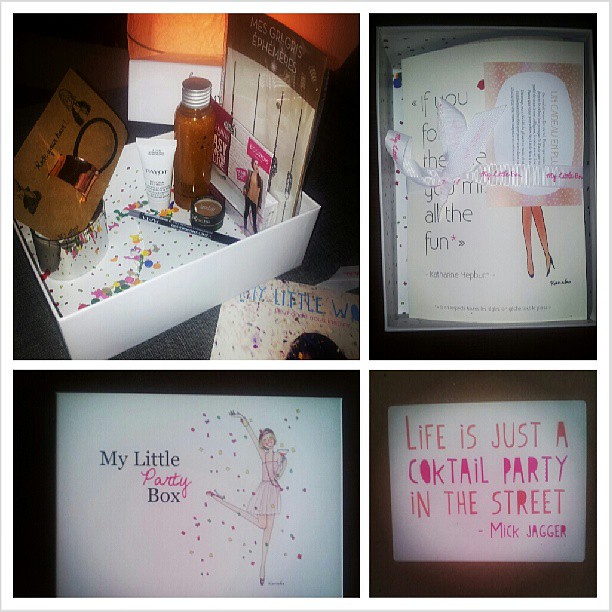This is a full-color collage composed of four separate photographs, arranged in a windowpane format. The top left image features a white box filled with a variety of items: a tube of cream, a glass container with a silver lid, an eyeliner pencil, a small round container possibly holding eye shadow, and multi-colored confetti. The top right image displays a drawing encased in a plastic protector, partially obscured by ribbons and other items. Visible text reads, "if you [...] all the fun." The bottom left image shows a rectangular box labeled "My Little Party Box" with a color pencil sketch of a woman in a pink dress, raising her arm as if she's sprinkling confetti while holding a drink. The bottom right image showcases a sign with a quote, "Life is Just a Cocktail Party in the Street" attributed to Mick Jagger. The collage features diverse hues including black, white, dark blue, pink, tan, purple, brown, green, blue, yellow, and orange, evoking a festive and vibrant atmosphere.